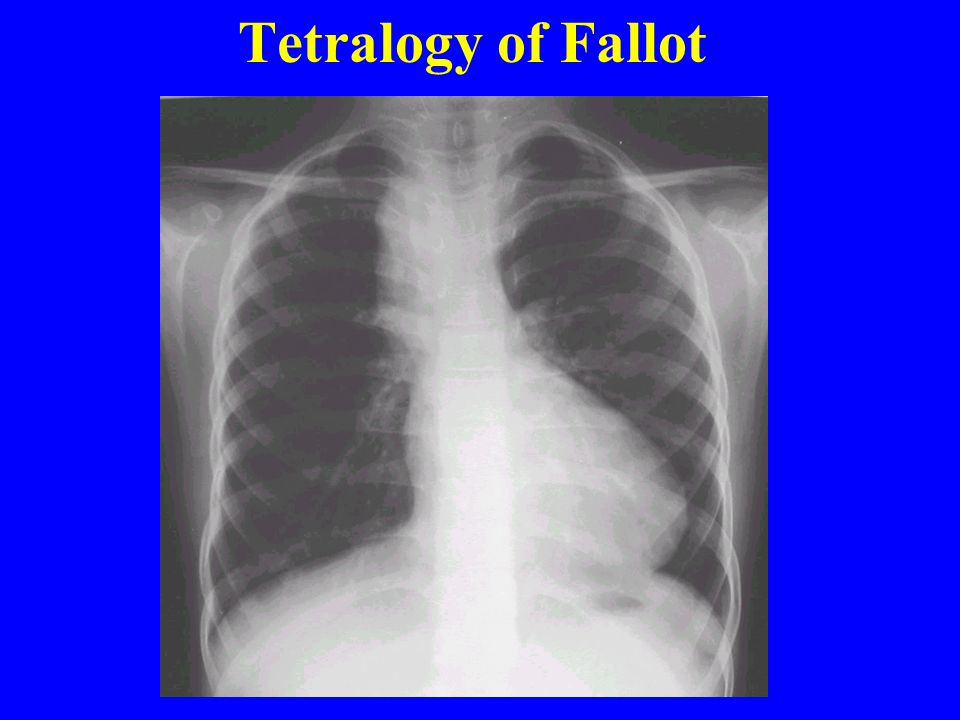The image is a medical presentation slide featuring a detailed x-ray of a person's chest, encased within a vivid blue background. Centered at the top, the text "Tetralogy of Fallout" is displayed in a bright yellow font, with capital letters T and F. This x-ray clearly depicts the intricacies of the ribcage, collarbone, and shoulder blades, revealing the white outlines of bones and organs contrasted against the black areas indicative of air-filled lungs. Notably, the heart is visible, protected by the ribs, while the spinal column and individual vertebrae are distinguishable. The clarity of the lungs suggests they are free from obstructive material, indicating healthy respiration.